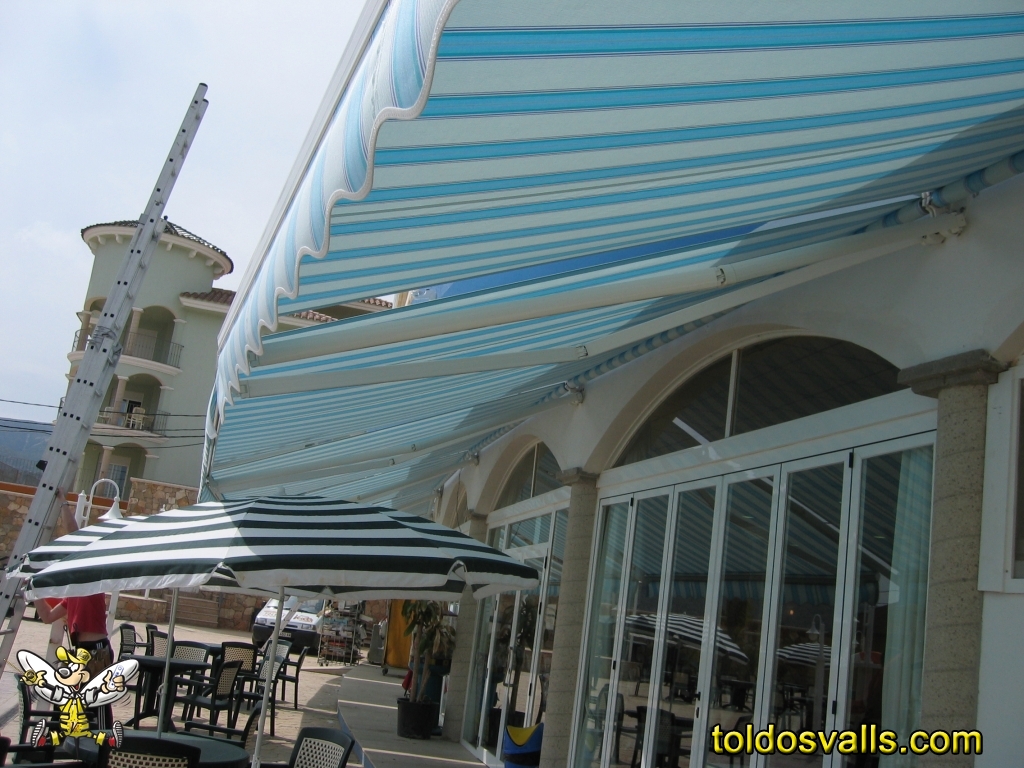This is a color photograph taken during the daytime, capturing a lively street scene from a sidewalk perspective. Prominently, a three-story building stands in the background, partly obstructed by a store in the foreground. The storefront features a striking blue and white striped awning that stretches down the sidewalk, complemented by blue and pink borders. Below the awning, a row of glass panels, separated by white dividers, reflects the urban bustle.

In front of the store, a patio area is set up with a black and white vertically striped umbrella shading a metal table, part of a trio of such sets. In the distance, to the right of the patio, a van is parked at the end of the row of umbrellas, adding to the city atmosphere. Additionally, just inside the frame's lower left-hand corner, a whimsical cartoon character resembling a bee in a hat adds a playful touch to the scene. The three-story house on the corner, recognizable by its tower-like structure and doorway shapes, completes the vibrant and detailed urban snapshot.